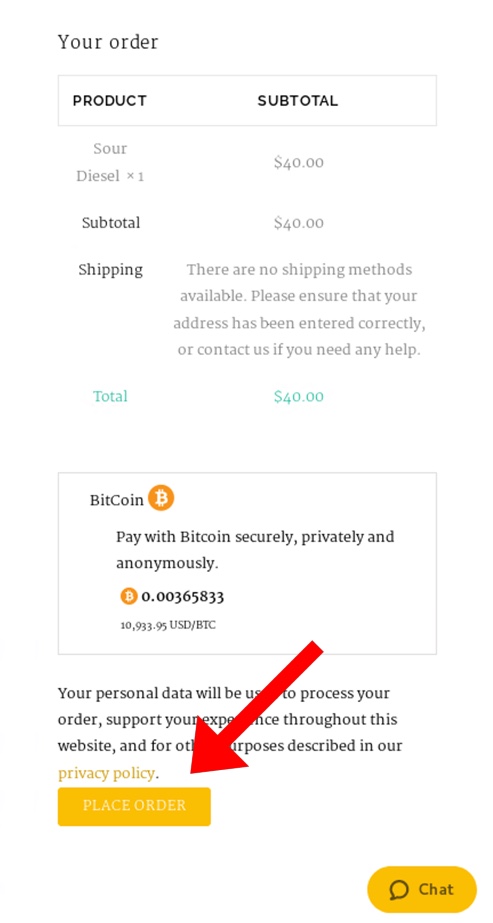**Screenshot Overview: A Breakdown of a Mobile Order Summary Page**

This portrait-oriented screenshot appears to have been taken on a mobile phone, displaying the order summary of an online purchase. The background is predominantly white, with black text making the content highly readable.

**Header Section:**
- At the very top of the screen, bold black text reads "Your Order," indicating this screenshot pertains to an ongoing or completed purchase.

**Order Details Section:**
- Below the header, there's a gray outlined box with a white background, containing two columns labeled "Product" and "Subtotal."
- The product listed is "Sour Diesel," with a quantity of "1."
- To the right of the product name, the subtotal amount is displayed as "$40."

**Shipping Information Section:**
- Just below the product details, the subtotal is reiterated.
- The shipping information states that no shipping methods are available. A note advises the user to ensure their address is correct or to contact support for assistance.

**Total Cost Section:**
- The total cost of the order is highlighted in a bluish-green font, clearly stating "$40."

**Payment Options Section:**
- Following the total cost, there's another gray outlined box featuring the Bitcoin symbol and the word "Bitcoin."
- This section outlines the option to pay securely, privately, and anonymously using Bitcoin. It includes the cost in Bitcoin and the current conversion rate.

**Call to Action and Support Section:**
- There is a prominent red arrow pointing from the Bitcoin payment box to a yellow "Place Order" button, partially obscuring a short message about the site's privacy policy regarding personal data.
- In the bottom right corner of the screen, another yellow button with black text offers a chat support option for additional help.

This detailed layout provides a clear and comprehensive view of the order summary, ensuring the user understands all aspects of their purchase and available options.